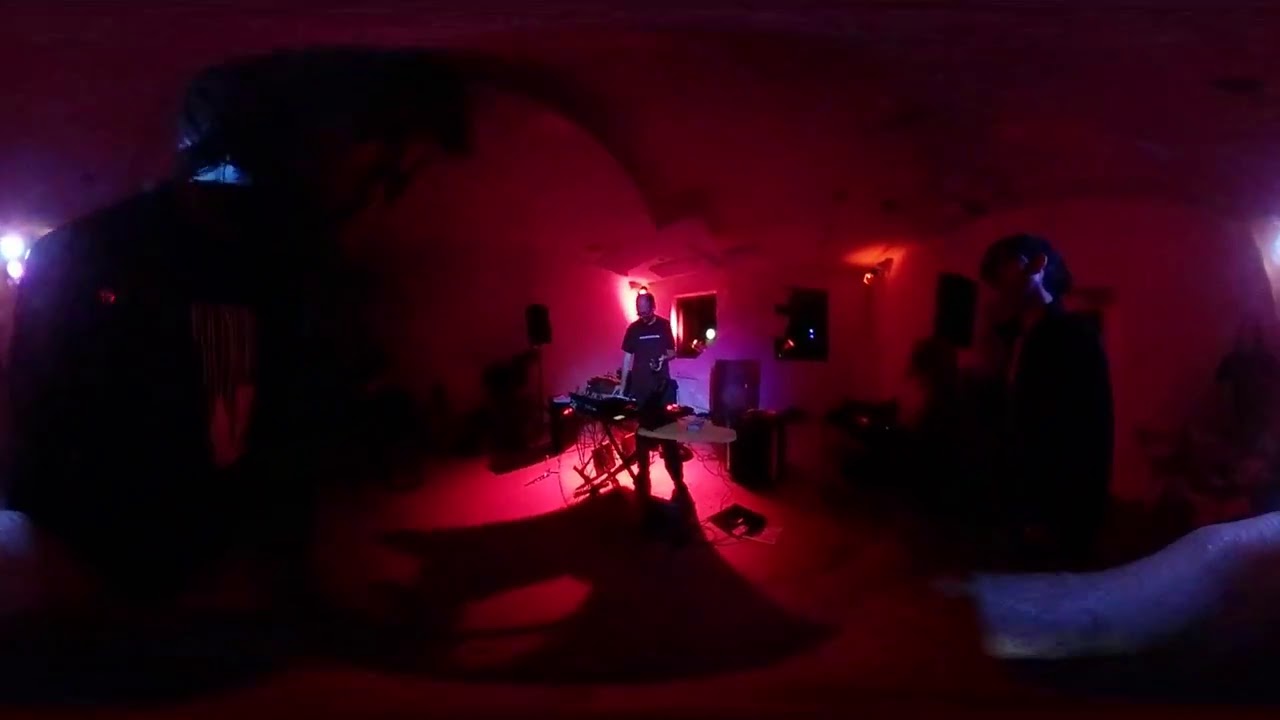In this intriguing and atmospheric image, we see a male figure presumably performing a DJ set in a dimly lit indoor space. The man's right hand is placed on a keyboard-like instrument, while his left hand rests at his waist. He is wearing a dark, possibly navy blue shirt with indistinct white lettering across the chest and has thinning hair on top of his head. The room features a unique circular and cylindrical distortion, creating a fisheye lens effect that emphasizes the man at the center while the surroundings curve dramatically back. 

The lighting in the scene casts a reddish-pinkish hue that brightens towards the center but darkens towards the edges, adding to the surreal ambiance. There is also a subtle blue glow illuminating the backs of faintly visible individuals on the periphery and behind the central figure. Windows are visible in the background, appearing square and set within lighter-colored walls, with the darkness outside indicating it is nighttime. On the floor near the individual, there are pieces of audio equipment, likely a speaker and amplifiers, which enhance the impression of a live performance in progress.